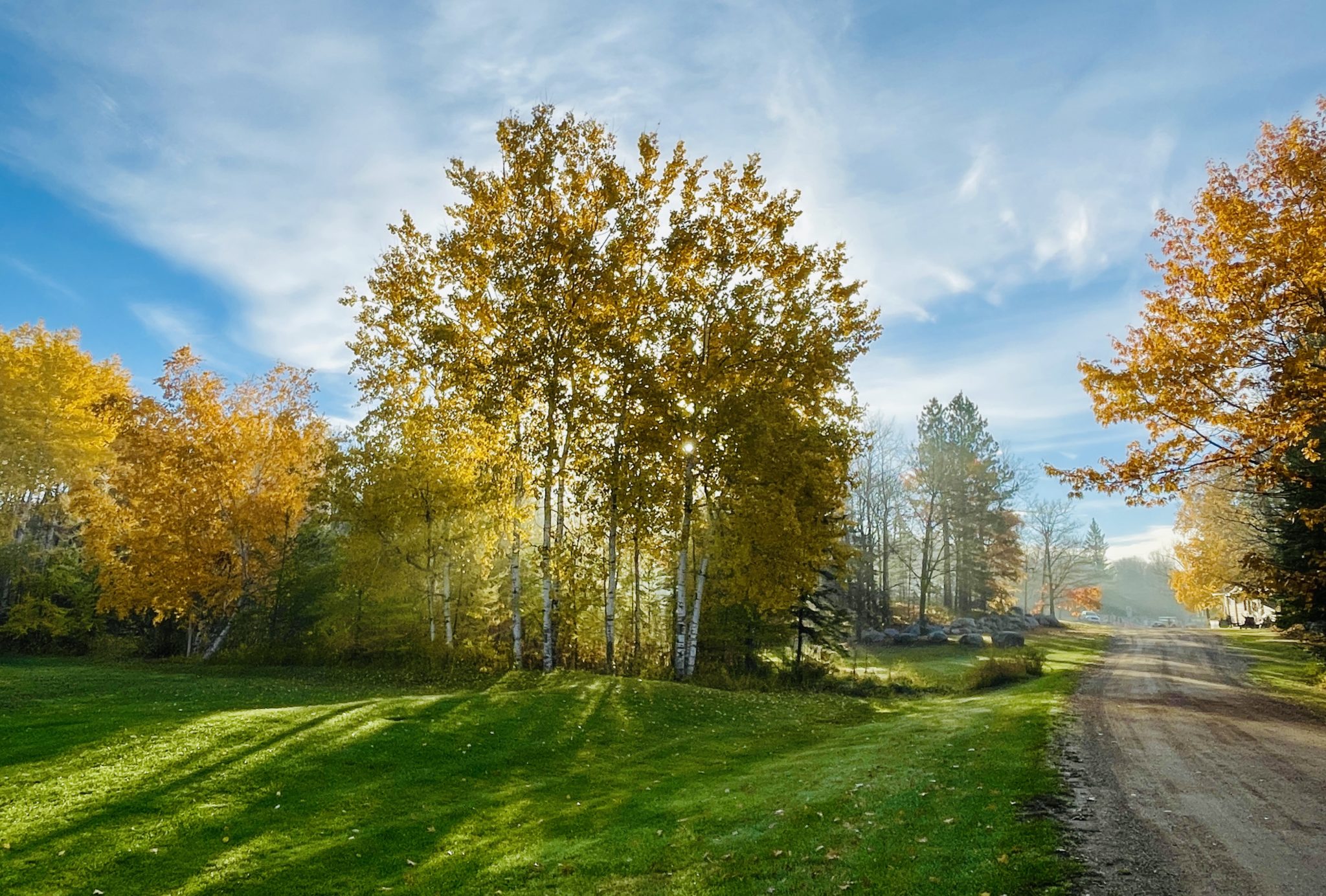The photograph, taken outdoors in the fall, features a captivating scene dominated by tall trees with golden leaves stretching towards the sky. In the center, sunlight streams through the trees, casting intricate shadows on the green grass below and highlighting the autumnal hues. To the left, additional trees, adorned in shades of gold and yellow, stand against a backdrop of a blue sky filled with wispy white clouds. Below these trees, a grassy field extends towards the horizon. On the right side of the image, a dirt road meanders into the distance, flanked by trees with leaves in various stages of changing colors, from green to brown to gold. Towards the end of the road, cars are parked near a white building partially obscured by more trees. Scattered leaves blanket the ground, and a series of rocks and a possible fence can be seen amidst some barren trees on the left side of the road, adding to the rustic charm of the scene. Overall, the image captures the serene beauty of a crisp fall day, blending vibrant foliage, a clear sky, and natural light to create a vivid depiction of the season.